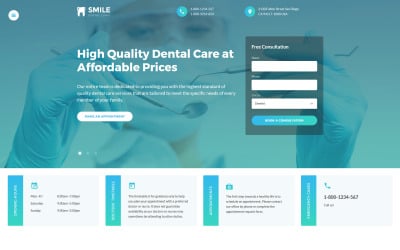The image depicts a page with a turquoise background featuring a blurry photograph of a dentist wearing natural-colored gloves, holding a dental mirror and a scaling tool, and donning a face mask. At the top of the page, the word "Smile" is prominently displayed. To the right, there is additional text that is difficult to decipher in the blurred image. Two lighter blue circles can be seen, one containing a phone icon and a set of numbers, while the function of the other circle remains unclear. The text "High-quality dental care at affordable prices" is visible beneath these circles. There is further text below this statement and a noticeable white button meant for interaction. The phrase "Free something" is partially legible, followed by three boxes, two of which are text boxes and the third a drop-down menu with a blue button below it. Further down are four gray boxes with text inside, each accompanied by a blue box on the left side.